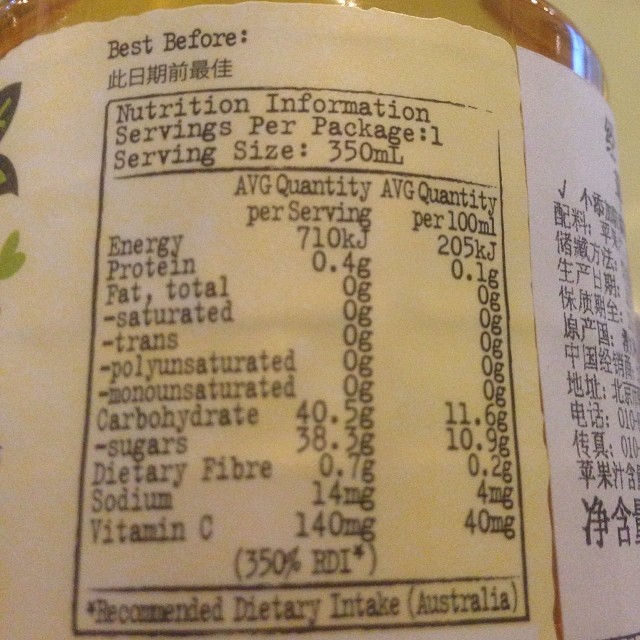This image captures a close-up of a label from a bottle or drink, likely an oil bottle, with both Chinese and English text. The majority of the label's text is in Chinese, including the best before date, while the main headings of the nutritional information and the numerical values are presented in English. The details indicate this product adheres to Australian dietary standards, suggesting it is marketed in Australia. Due to the high carbohydrate and sugar content, the product seems to be a sugary beverage. Given the substantial vitamin C content, it could be either an orange juice or a sugary, fizzy orange drink. The image's close-up nature obscures the rest of the bottle, preventing a precise identification of the product.